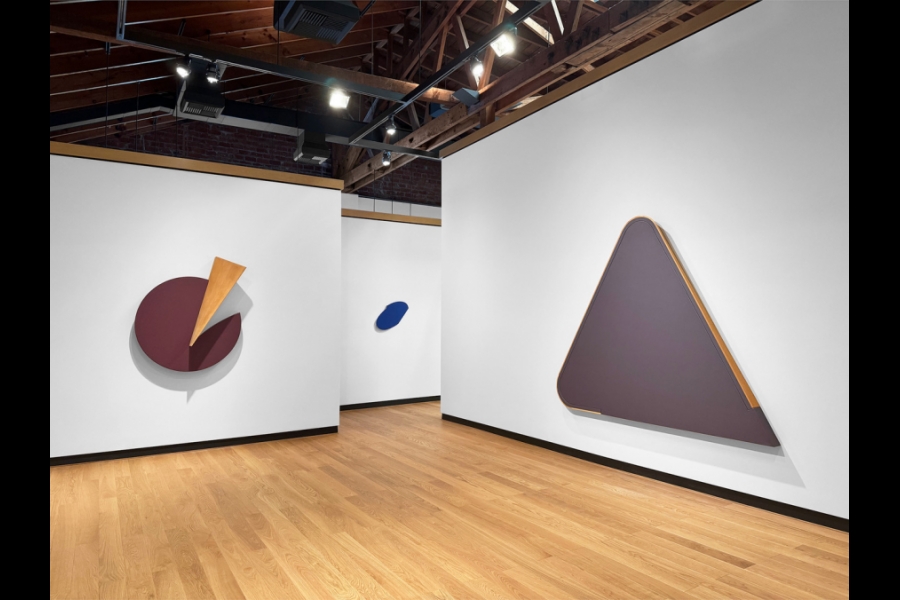The image depicts a clean and modern art gallery with a wooden floor and overhead lighting, featuring geometric abstract artworks against white walls. On the left is a predominantly maroon-colored, off-center circle resembling a pie chart with some of the sections missing, including an orange slice and a gray slice; it has a small point sticking out and an indistinguishable number that appears to be "2." In the center background, there's a skewed elliptical dark blue shape. On the right, a mauve triangular piece with one sharp edge and two rounded edges hangs on the wall. The gallery has a sophisticated ambiance with metal beams and wooden ceiling rafters, enhancing the presentation of the art.